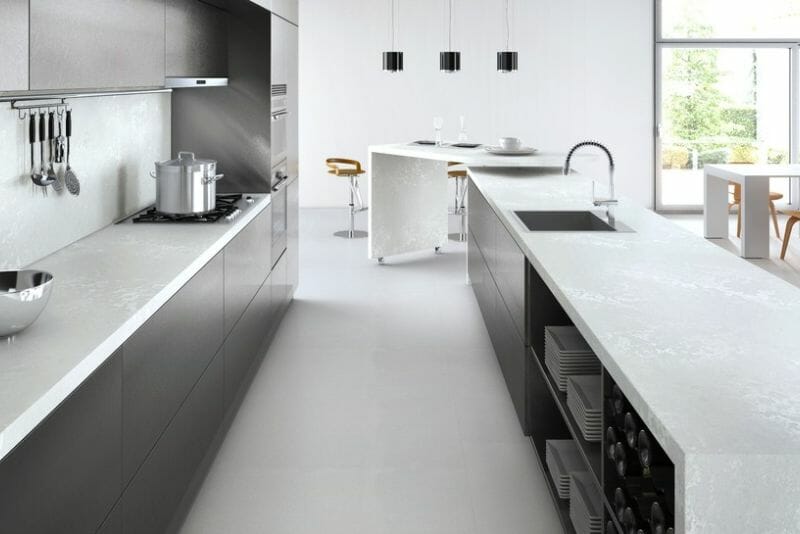The photograph captures a large, modern kitchen primarily decorated in white and gray tones. The kitchen features sleek gray cabinets with a white marble countertop. On the left side, built into the cabinetry, is a stove with a silver pot placed on it and a rack above it holding various hanging spoons. Adjacent to the stove is a mixing bowl on the counter. The center of the kitchen is dominated by a rectangular island with white countertops, which houses a sink and a chrome faucet. This island also has storage underneath, including neatly stacked white, rectangular plates. 

Towards the back of the room, there is a dining area featuring a white table, surrounded by bar stools with brown and chrome finish. Above the table hangs black pendant lighting with three bulbs. On the right side of the room, there is another white table. The room is well-lit by a large floor-to-ceiling window or patio door, allowing ample daylight to stream in and offering a view of the outdoors, contributing to the kitchen's airy, stylish ambiance.